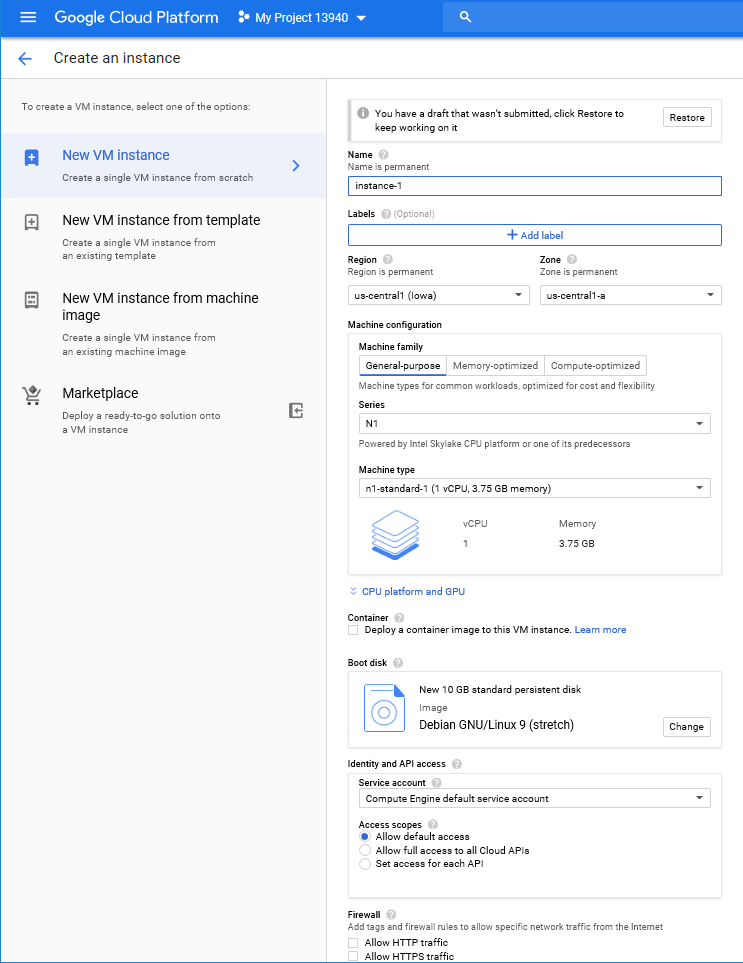The image appears to be a screenshot from a tablet showing an interface of the Google Cloud Platform. At the top, there is a blue band containing a menu icon with three horizontal white lines and the text "Google Cloud Platform" also in white. Next to it, there is the label "My Project 13940" with a dropdown arrow beside it and a search bar.

Below the blue band, the screen has a white background with a blue left-pointing arrow and the text "Create an instance" written in black. There is a menu or dropdown list open with several options: "Marketplace," "New VM Instance," "10 machine," "Instance from machine image," "New VM instance from template," and lastly "New VM instance" again. The "New VM instance" option is highlighted in blue, indicating it is selected, while the other options are listed in black.

On the right side of the interface, there is additional text in black, likely providing further instructions or settings related to the creation of the new VM instance. The detailed options and text guide the user through the creation process of a new virtual machine instance within the Google Cloud Platform.